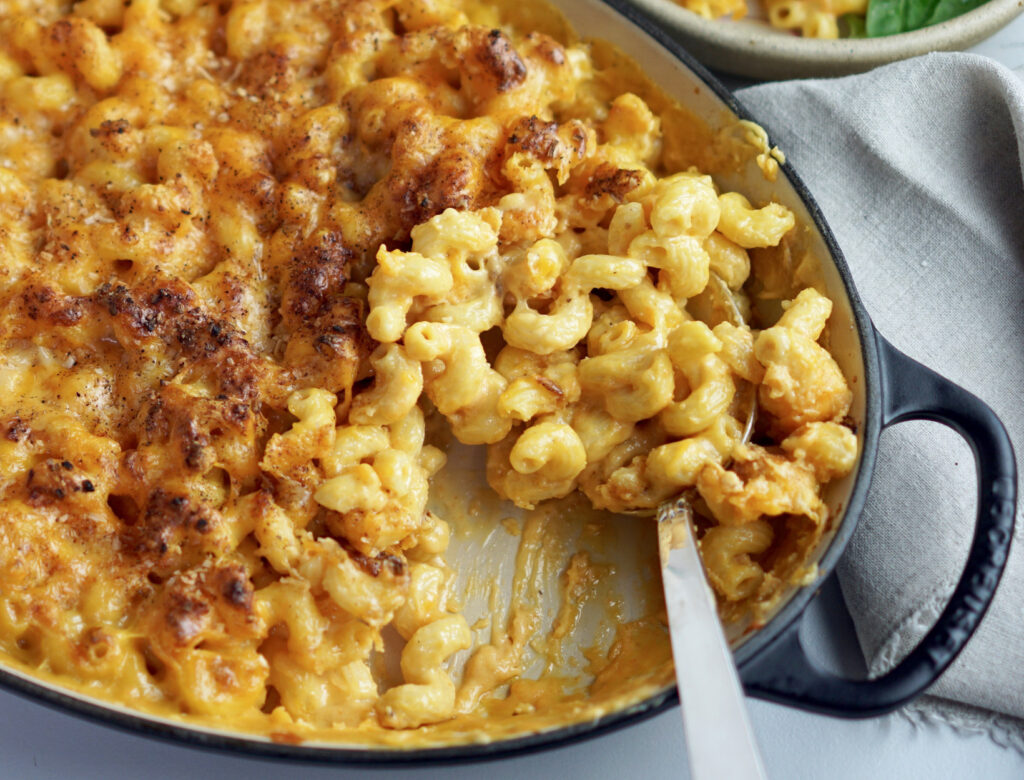This color photograph, taken in landscape orientation, captures a tantalizing view of a creamy macaroni and cheese casserole. The centerpiece is a large, black oval baking dish with a black handle emerging from the bottom right corner, angled slightly toward the top left. The interior of the dish is white, and the macaroni and cheese boasts a golden-brown, crusted surface, indicating a perfect bake. A silver serving spoon, partially buried in the casserole on the right side, suggests a recent serving with a portion visibly scooped out, revealing its gooey, creamy texture beneath the crust. The dish is placed on a gray surface, complemented by a gray napkin positioned at the bottom right corner. In the background, at the top right of the image, there is a smaller bowl also containing macaroni and cheese. The overall scene is set upon a gray linen cloth that enhances the dish's rich colors and textures, embodying photographic realism and appetizing food photography.